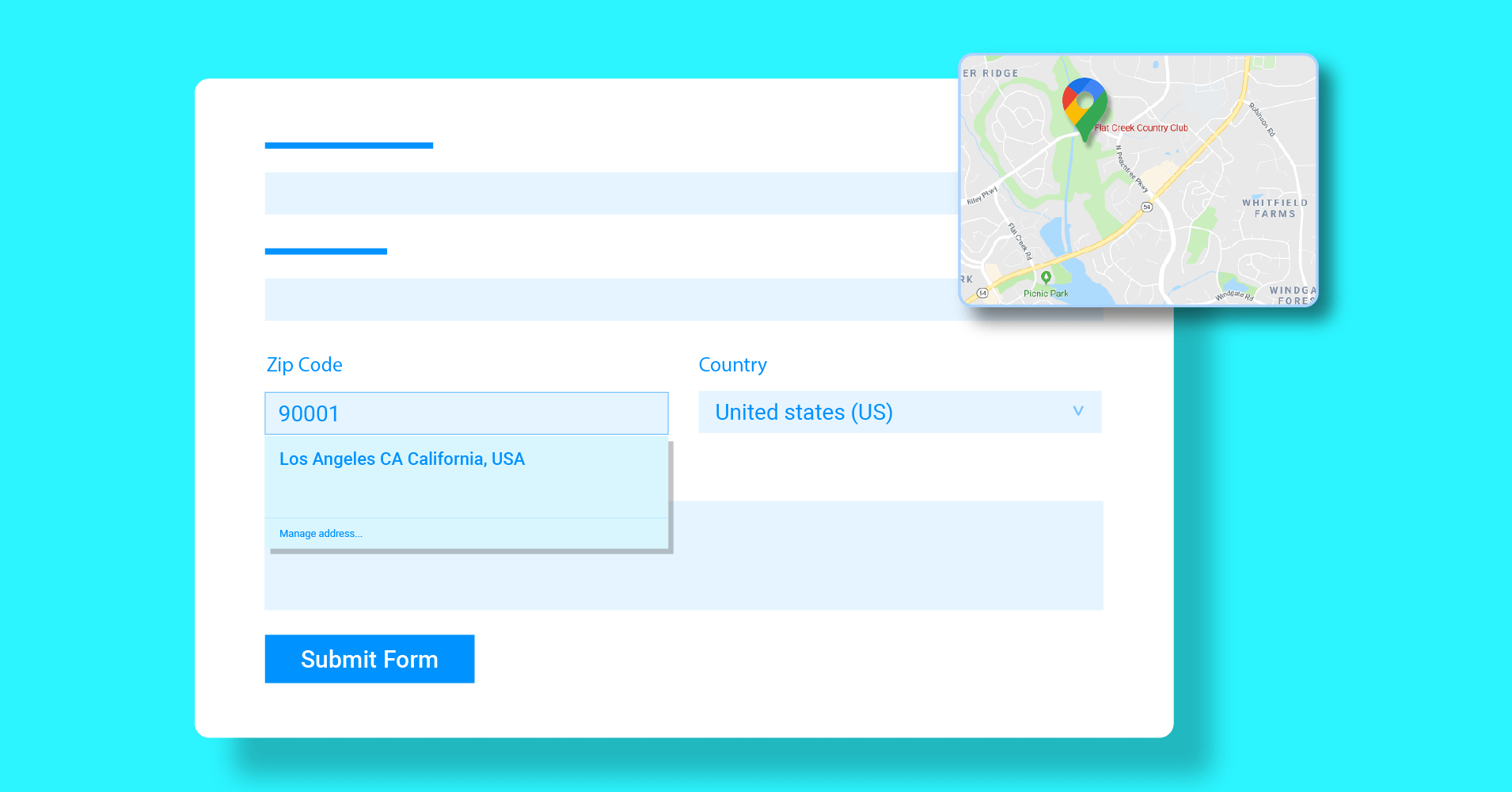This is a screenshot of what appears to be a Google Map interface, set against a striking background in a fluorescent Tiffany blue hue. The background color is vivid, almost luminescent. The main feature of the image is a white rectangular search bar at the forefront, designed for address input. Inside this bar, there are two royal blue lines framing entry fields, matching the text within which is also in royal blue. 

Beneath these entry fields is a royal blue button labeled "Submit Form." The initial two input boxes are empty, while a third field designated for the zip code is populated with "90001," resulting in the location identified as Los Angeles, California, USA. Additionally, a country selection box displays "United States (US)."

Accompanying this interface is a map pinpointing the input zip code, with a recognizable Google Maps marker highlighting a green area labeled "Flat Creek Country Club." The overall design is both functional and visually appealing, merging practical map elements with distinctive color choices.